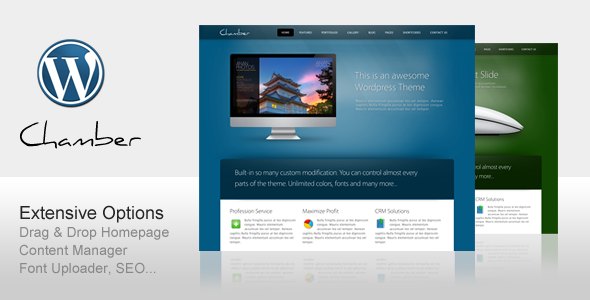The webpage features a mid-gray background. On the left side, there is a dark blue circle with a matching dark blue interior and a white band encircling it. Inside the circle is a stylized 'W', with a small, bubble-like embellishment on the right side of its end. Below this emblem, the word "CHAMBER" is written in a black, chalk-like font.

Underneath this section lies a lighter gray rectangle, containing bold black text that reads "Extensive options." In dark gray text beneath it are the phrases: "drag-and-drop homepage, content manager, front uploader, SEO..." 

Central to the layout is a dark blue bezel showcasing several clickable tabs, with one tab currently selected. Within a dark blue area, highlighted by bands of white, there is a silver-bezeled monitor, possibly an Apple Macintosh, characterized by its silver vase and black bezel at the top. The monitor displays an image of a Japanese temple featuring brown rooftops and white walls.

Across a dark blue rectangle in the center of the screen, thin white text reads, "Build-in so many custom modifications, you can control almost every part of the theme." It further emphasizes, "Unlimited colors, fonts, and many more."

On the right side of the webpage, a dark green background hosts white text alongside a leaf-like graphic, accompanied by additional clickable tabs. There is also a darker green text box containing black text, although the specific content of this text is difficult to discern from the description provided.